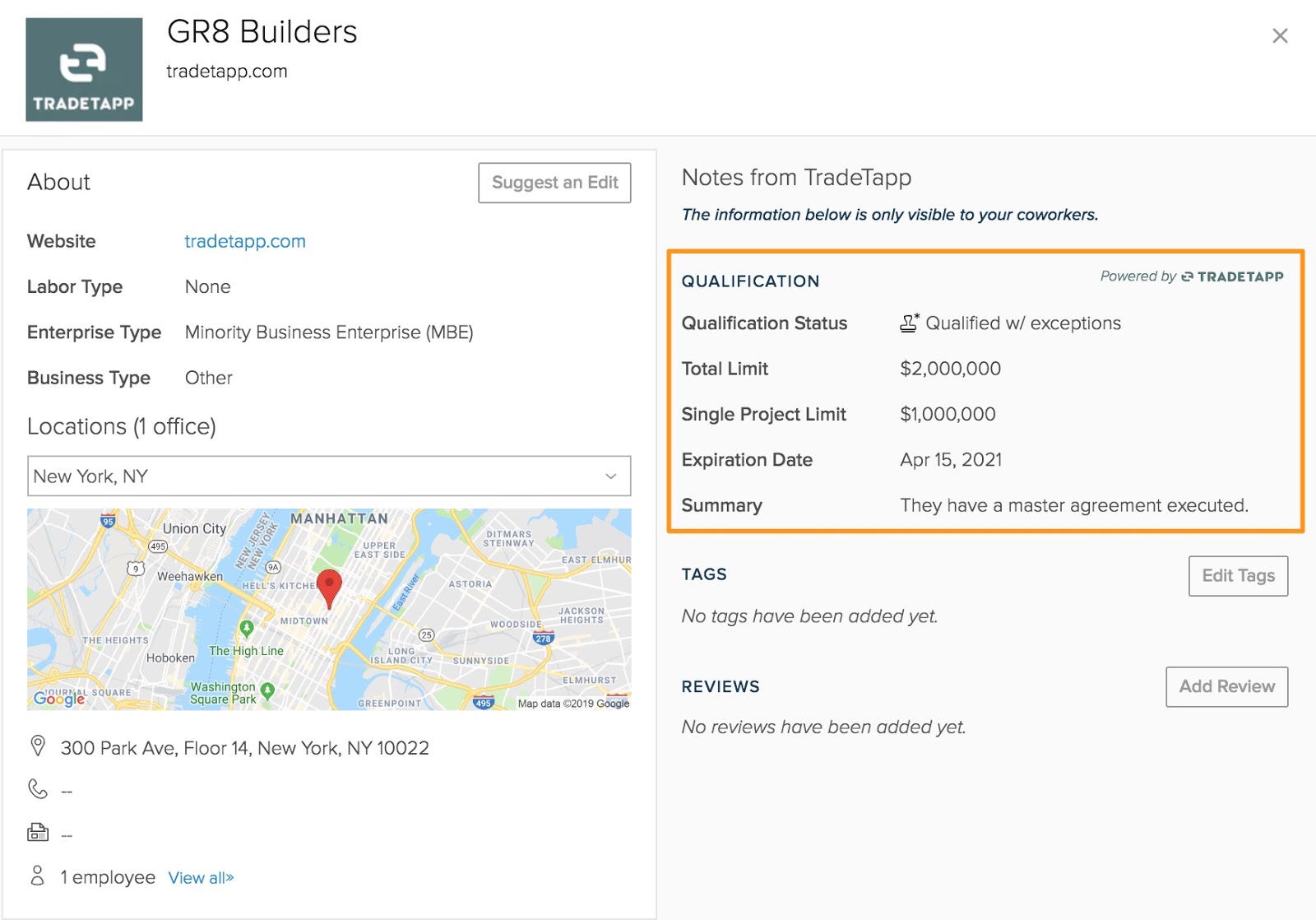The image captures a screenshot from the website TradeTap.com, featuring a detailed profile of the company GR8 Builders. The TradeTap logo is prominently displayed in white against a greenish background at the top of the page. Below the header, the website address is clearly marked as TradeTap.com.

The profile details of GR8 Builders are laid out as follows:
- Enterprise Type: Minority Business Enterprise (MBE)
- Business Type: Other
- Location: Office in New York, New York

A Google Map is embedded, highlighting the office location with a red marker. The full address is:
300 Park Avenue, Floor 14, New York, New York, 10022.

Additional profile information includes:
- No telephone number
- One employee (with a clickable link to "view all" in blue)

On the right side, there is a section titled "Notes from TradeTap," indicating that the information below is only visible to coworkers. Key qualifications are:
- Qualification Status: Qualified with Exceptions
- Total Limit: 2 million
- Single Project Limit: 1 million
- Expiration Date: April 15, 2021
- Summary: Master Agreement Executed

There are also sections for tags and reviews, both currently empty. The overall impression is that this is a report card-like summary of GR8 Builders' qualifications and status on the TradeTap platform. No further information is provided.